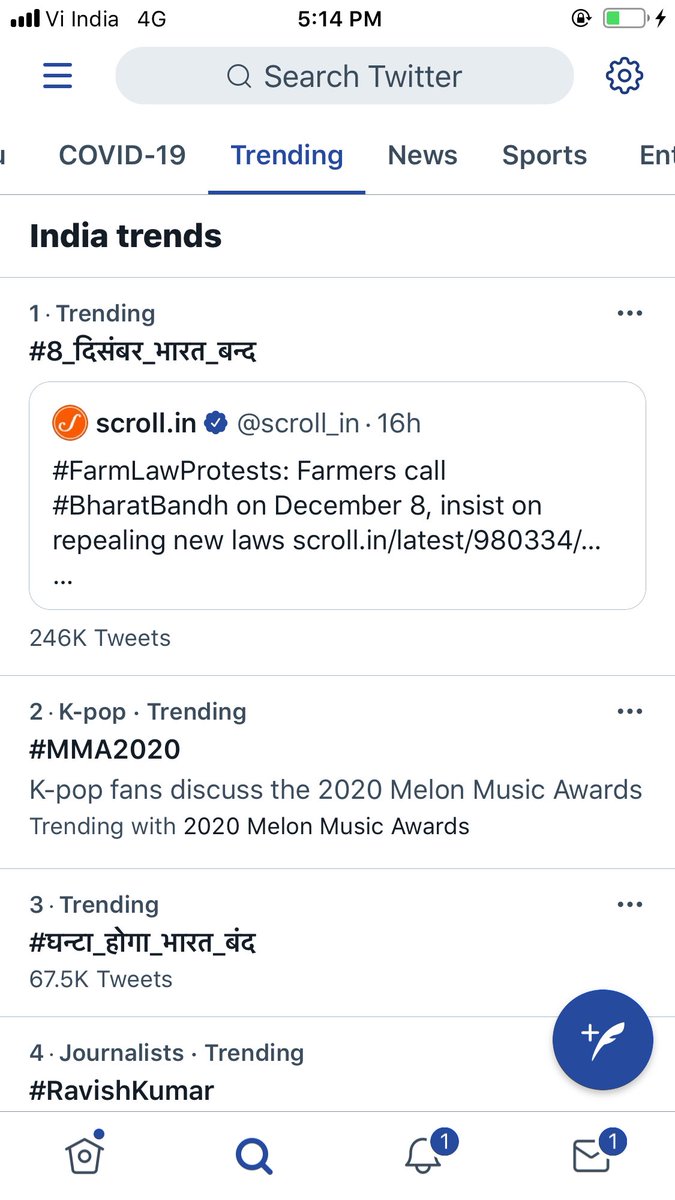The image displays a Twitter trending page on a mobile device. The status bar at the top shows a full network signal from VI India with 4G connectivity, the time, a screen orientation lock icon, and a battery charging indicator. Below the status bar, there's a search field with a magnifying glass icon and the placeholder text "Search Twitter." To the right of the search field, a settings icon is visible. The content below includes various trending topics such as the COVID-19 pandemic, news, sports, and specific trends from India, including ongoing farm law protests with hashtags like "Bharat Bandh on December 8th" and calls to repeal certain laws. Additionally, a trend about K-pop fans discussing the 2020 Million Music Awards is noted, linked with the hashtag "2020 Million Music Awards."